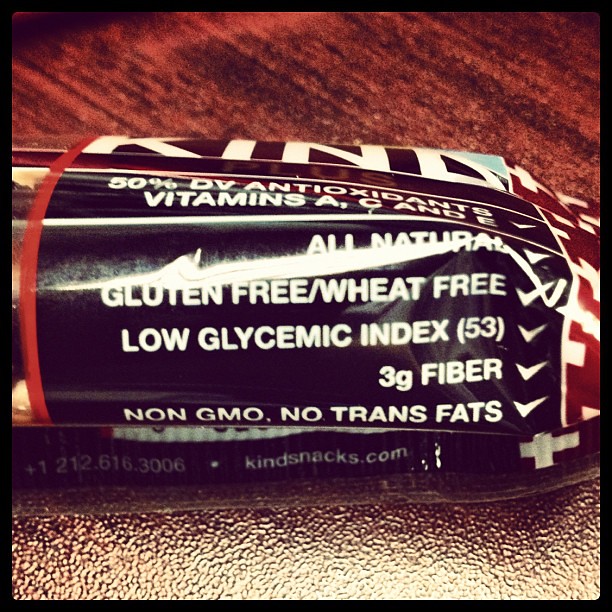In this photograph, a food item resembling a sausage is prominently displayed on a rustic brown wooden table. The sausage-like product stretches horizontally across the entire frame, its right end showing a discernible curve, enhancing the perception that it might indeed be a sausage. The product is encased in a label that is predominantly black with white text, indicating a brand called "KIND". The label highlights several health benefits: "50% more antioxidants," "Vitamins A, C, and E," "All natural," "Gluten-free," "Wheat-free," "Low glycemic index of 53," "3 grams of fiber," "Non-GMO," and "No trans fats." At the bottom of the label, there is a lot number alongside the website "kindsnacks.com," suggesting the authenticity and traceability of the product.